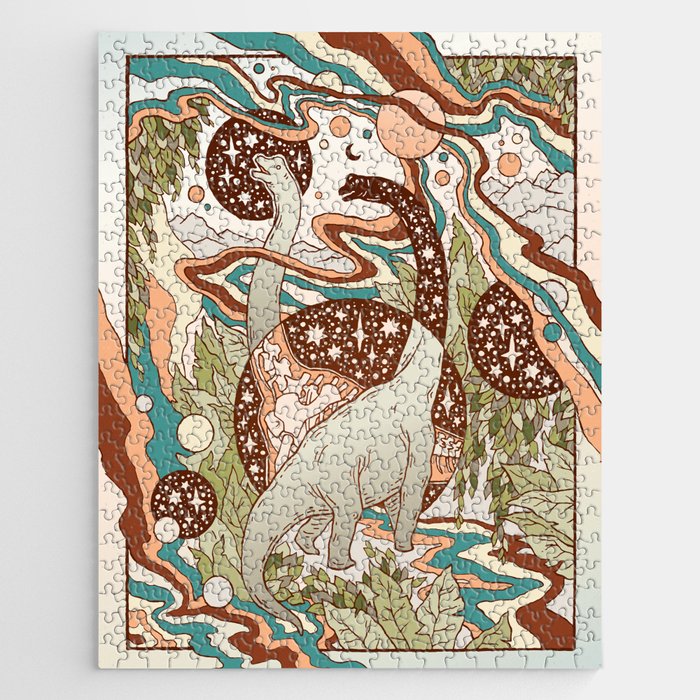This image is a highly detailed and colorful photograph of a completed jigsaw puzzle set against a white background. The puzzle forms a vertical rectangular artwork featuring two relaxed brontosauruses surrounded by an intricate blend of natural and celestial elements. The prominent colors in this piece are a rich tapestry of blues, greens, browns, tans, burnt sienna, sage greens, and touches of pink and purple.

The dinosaurs are depicted with their long necks elegantly arching, one looking to the left and the other towards the sky. Their gray bodies are accentuated with dark brown trimming, and there's an artistic use of circles and stars throughout, suggesting a celestial theme. Notably, within a large circle in the middle, there is an x-ray-like cross-section showing the skeletal structure of the dinosaurs, rendered in a stark black filled with stars.

The background combines natural foliage like trees, bushes, and vibrant green leaves with more abstract elements. Wavy lines in varied colors—turquoise, red, peach, and off-white—create a dynamic, flowing pattern around the dinosaurs. Several large and small spheres of different colors, possibly representing celestial bodies like the sun and moon, dot the scene. These elements overlap with strips of mist winding around the dinosaurs’ necks.

Adding to the artistic complexity, there is a noticeable white border around the puzzle, where the indentation lines of the individual pieces are visible, emphasizing that this is a jigsaw puzzle. The backdrop is lighter on the right and darker on the left, hinting at a gradient effect and giving the overall image a realistic and multidimensional feel. The puzzle seamlessly blends the natural and the fantastical, making it a captivating visual piece.